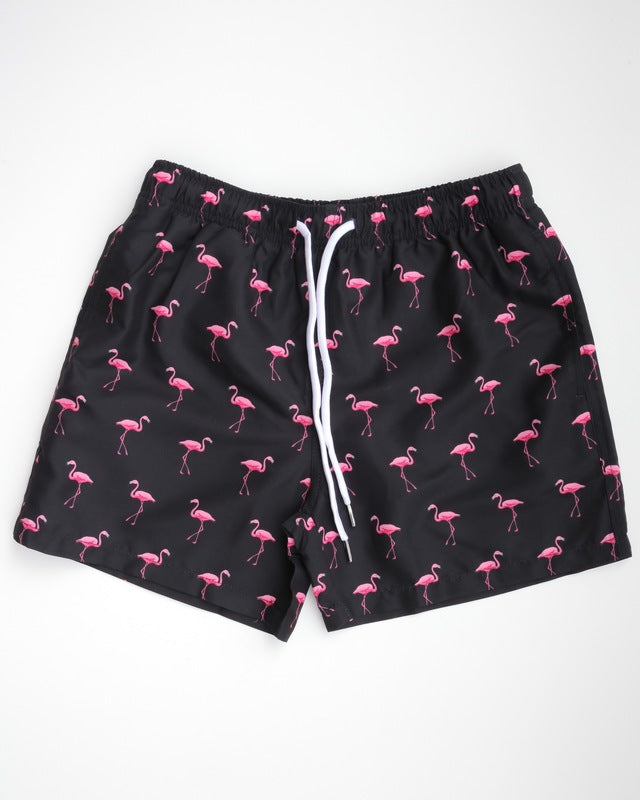This is a detailed photograph of a pair of men's swim trunks displayed against a light grayish lilac background that fades to almost white at the bottom. The swim trunks are black with a pattern of pink flamingos arranged in alternating directions. Each row of flamingos faces opposite to the one above and below it, creating a striking and playful design. The trunks are relatively short, not extending far below the crotch area, and are equipped with an elasticized waistband. Two white drawstrings with aglets dangle down the front from this waistband, reaching a considerable length along the shorts. The clear, vibrant details suggest these trunks are designed for swimming, characterized by their snug fit and eye-catching pattern.